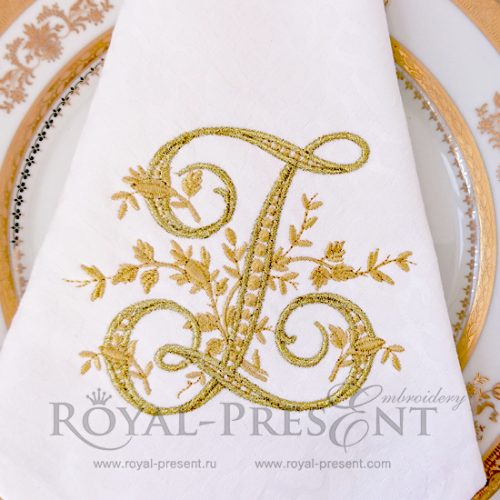The image is a professionally photographed advertisement showcasing an elegant dining setup. Central to the image is a large, round, white dining plate with intricate golden designs and a refined golden ring at its perimeter. Inside this golden ring are small, red shapes arranged in a circular pattern, adding a touch of contrast to the luxurious design. Resting atop the plate is a white cloth napkin, exquisitely embroidered with a large, gold, cursive letter 'L'. Surrounding the letter are delicate golden leaves and branches, enhancing the sophisticated aesthetic. Beneath the napkin, at the bottom of the image, the text "Royal Present Embroidery" is displayed in light gray font, with the second 'E' in 'Present' and the 'E' in 'Embroidery' capitalized and stylized. Additionally, two website URLs, www.royal-present.ru and www.royal-present.com, are listed, emphasizing the image's promotional nature. The overall composition of the image is square, viewed from a top-down perspective, and effectively conveys a sense of luxury and refinement.